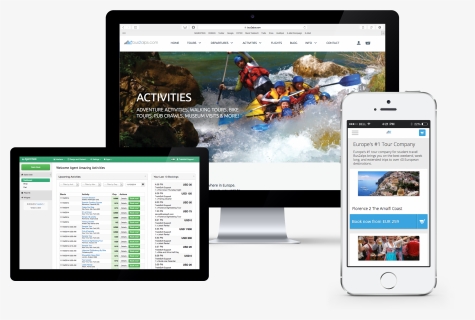The image consists of three distinct sections, each showcasing different technological devices. The main focus is a large rectangular gray background that serves as a backdrop for the other elements.

To the lower left, there is a black tablet with a white screen displaying an organized layout. At the top of the tablet screen, there's a green-bordered section followed by several columns. On the far right side of the tablet screen, numbers are visible, and a vertical series of green buttons appears towards the middle.

In the background, there's a computer monitor with a black exterior. The screen features an engaging graphic of people white-water rafting in a small raft amidst turbulent waters. Next to this image, the word "activities" is prominently displayed on the left. The upper portion of the monitor screen comprises a gray and white area segmented into various tabs and columns, suggesting a navigational or informational interface.

On the right side of the image, a silver phone is visible with a pop-up on the screen. This pop-up contains an image of a rocky mountain under a partially cloudy blue sky. The top of the pop-up includes a heading referring to "Europe's number one tour company," while the lower portion displays another picture, likely part of an advertisement for booking tours and activities through the company.

Overall, the image depicts a harmonious blend of devices and interfaces used for planning activities and tours, providing a comprehensive visual representation of interactive and informative technology in action.